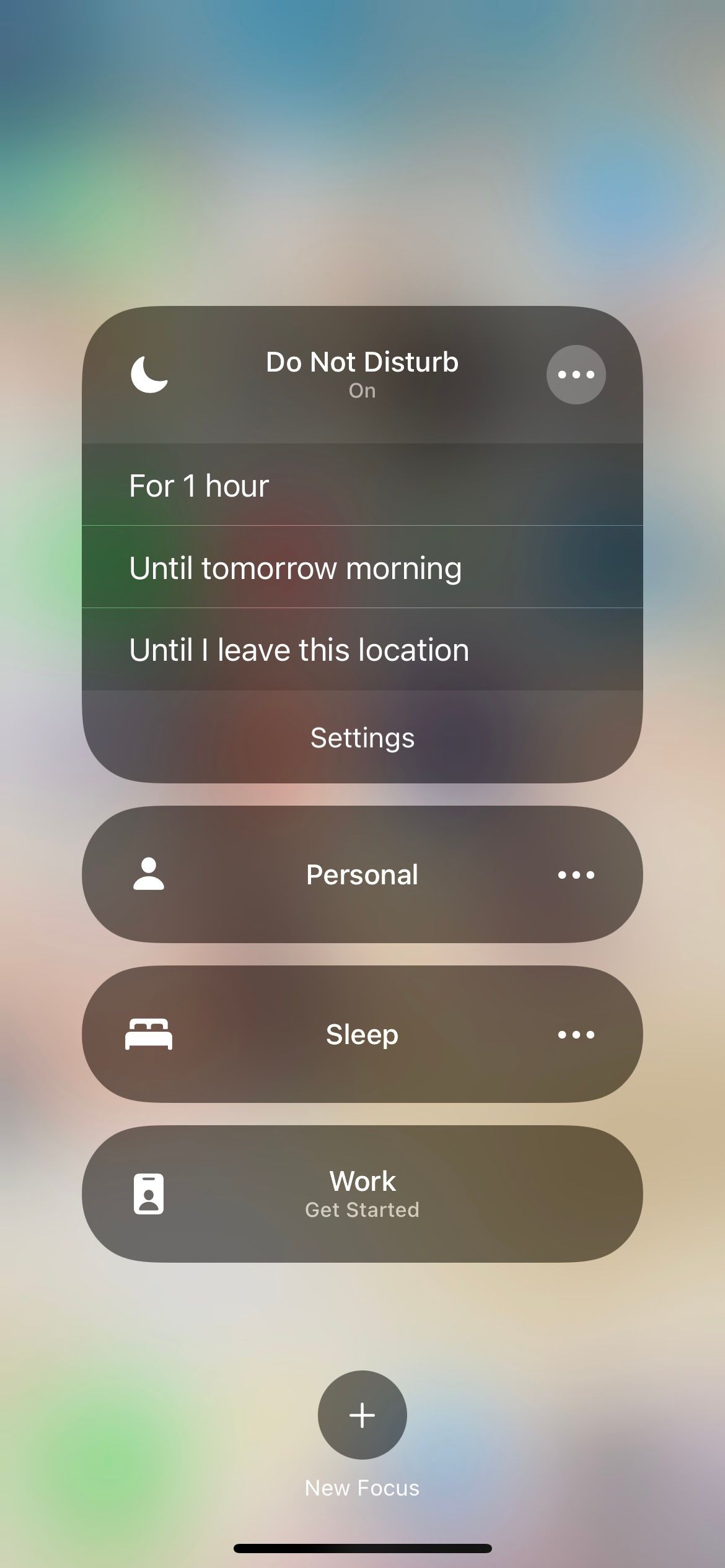The image is a screenshot taken from a smartphone, where the background is blurred to focus on the overlaying rectangles that have appeared on the screen. At the top, there's a brownish, curved-edged rectangle displaying the "Do Not Disturb" feature, with a moon icon in the upper left corner and a circle containing three horizontal dots. It indicates that the "Do Not Disturb" mode is turned on, offering options to remain active for one hour, until tomorrow morning, or until the user leaves the current location. Below this, a "Settings" option is visible.

The subsequent overlapping rectangle features an icon of a person and is labeled "Personal," accompanied by three horizontal dots on the right. Another rectangle below it, displaying a bed icon, is labeled "Sleep," also including the three-dot menu.

Further down, there's a rectangle labeled "Work," with an icon resembling a work badge, and a "Get Started" prompt. Below all these rectangles is a brown circle with a white plus sign, labeled "New Focus," indicating the option to add a new focus mode. Finally, a black line marks the bottom edge of the screen.